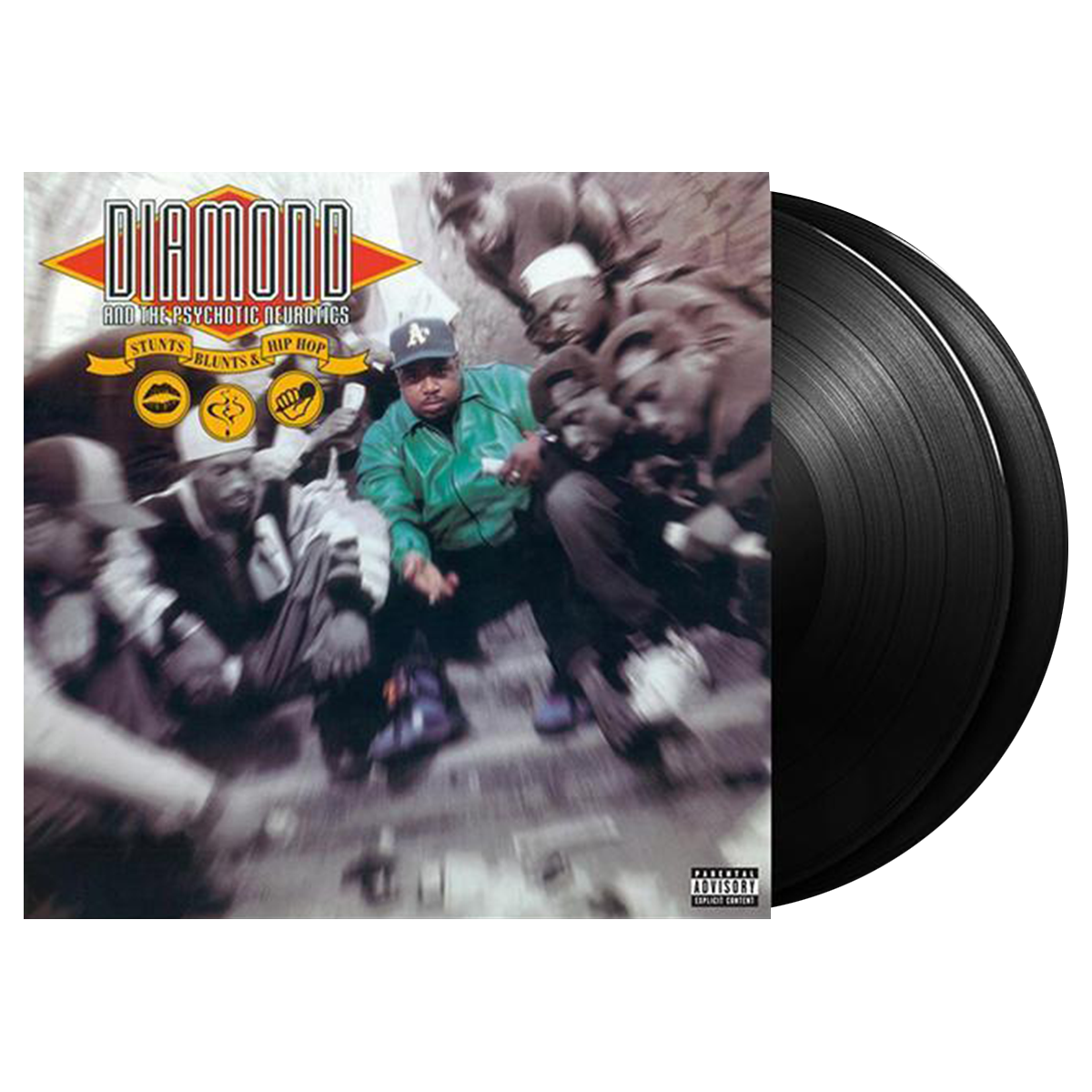The image features a square-shaped album cover, approximately four inches high and wide, set against a plain white background with no visible borders. Emerging from the right side of this cover are two black vinyl records. The central illustration on the cover portrays a group of African-American men engaged in a dice game, with most of them rendered in black and white. The pivotal figure, positioned centrally, contrasts the rest with vibrant coloration—he wears a black baseball cap adorned with a white letter 'A', a green leather zip-up jacket, and black pants. His hand extends forward, emphasizing the act of rolling dice, while he sits on steps.

The album cover's design includes a red diamond with a yellow outline in the upper left-hand corner, bearing the black-printed and white-outlined text "Diamond and the Psychotic Neurotics." Beneath this, a gold banner with black lettering displays the album title, "Stunts, Blunts, and Hip Hop." Three gold circles are arranged below, each containing distinct icons: black kissy lips in the first, smoke plumes from a cigar in the second, and a hand gripping a microphone in the third. In the lower right-hand corner, the phrase "Parental Advisory Explicit Content" is inscribed in black and white. This vivid cover encapsulates a dynamic scene while distinctly showcasing the album’s title and artist.